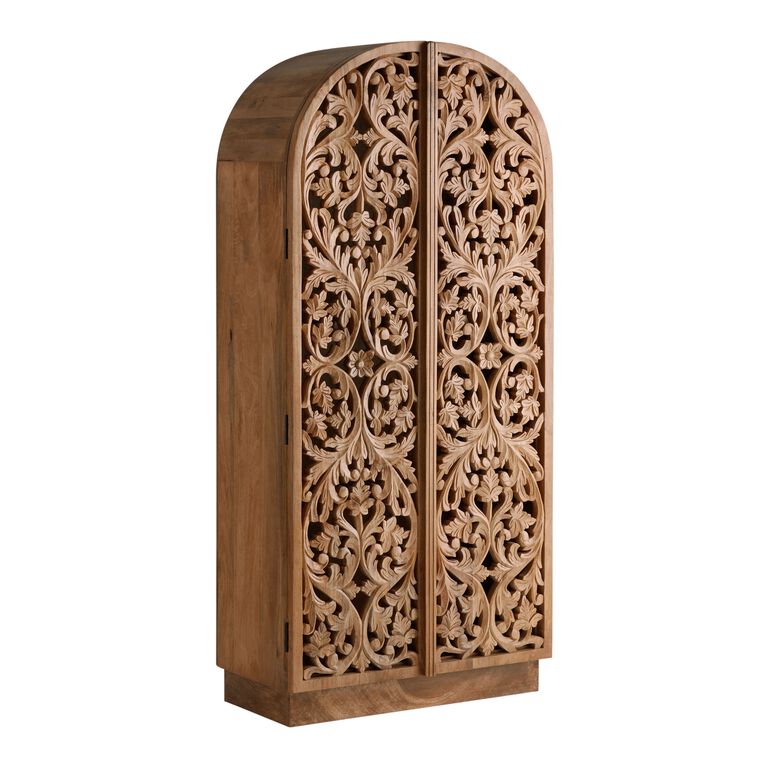This image showcases a detailed photograph of a tall, standing wooden cabinet set against a plain white background. The cabinet, characterized by its rich dark brown finished wood, features a distinctive design with its box-shaped lower section and a curved, rounded top. It stands on a slightly narrower base, providing stability and an aesthetic balance. The cabinet boasts two intricate double doors, each adorned with elaborate carvings of swirling vine and leaf patterns, which are cut through the wood, adding depth and texture. These detailed carvings are symmetrical across both doors, except for the central vertical separation that includes two parallel vertical lines etched into a vertical wooden piece. The cabinet is further detailed with black hinges, adding to its vintage charm. Every inch of this piece, from its floral and leafy patterns to its overall design, reflects a high level of craftsmanship.